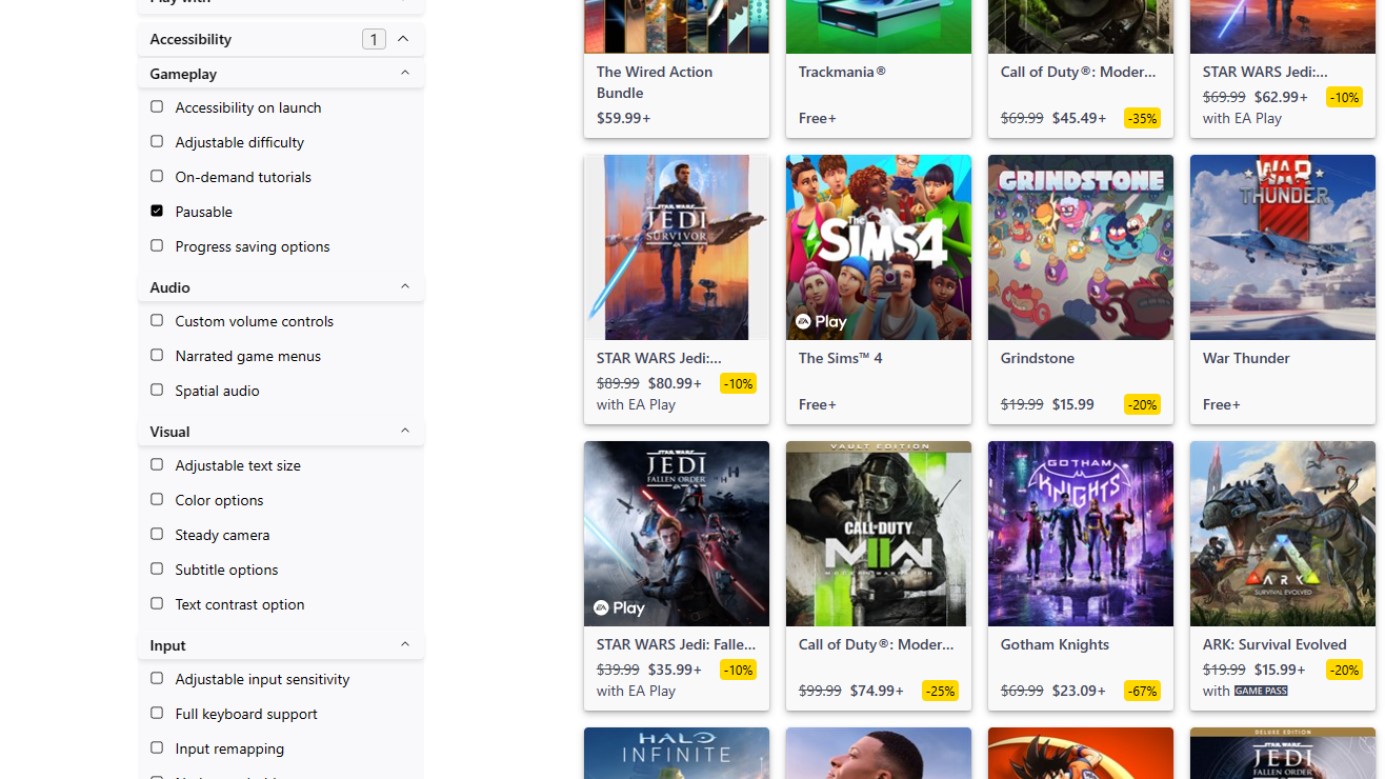A screenshot portrays an online gaming storefront interface offering a wide array of video games available for platforms such as PlayStation, Xbox, and PC. Prominently on the left side, a gray sidebar features a drop-down menu named "Accessibility," which is further divided into categories like Gameplay, Audio, Visual, and Input. The Gameplay section is expanded, displaying options such as 'possible highlighted.' 

In the main display area, a neatly organized grid exhibits 16 game titles. Key titles include "Wired Action Bundle" priced at $59.99, and a notable collection of four Star Wars games, including "Jedi." Other prominent titles are "Call of Duty: Modern Warfare," "Gotham Knights," "ARK: Survival Evolved," "War Thunder," "Grindstone," "The Sims 4," "Trackmania," and "Halo Infinite." Each game listing is accompanied by a visual thumbnail, though some titles are partially obscured.